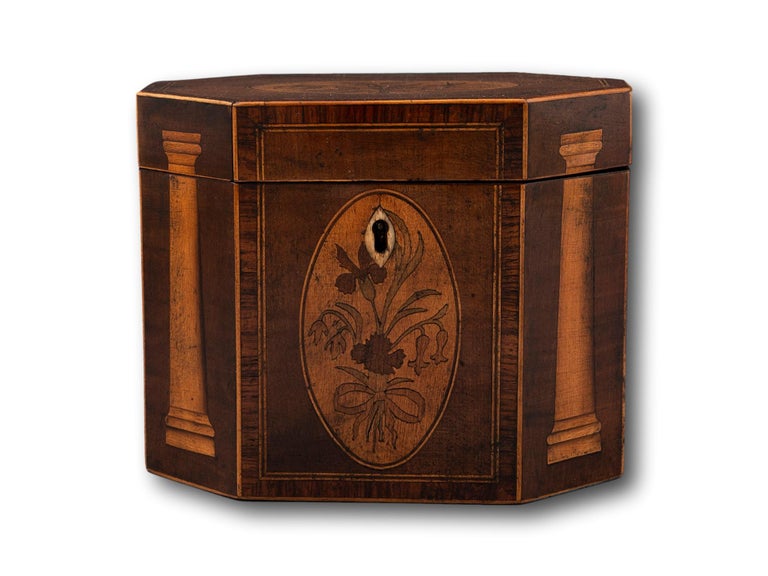The image depicts an intricately designed, dark brown wooden lockbox with an octagonal shape. The edges of the box are lined with light brown wood, emphasizing its geometric structure. Although the box appears to be resting on a white background, the primary focus is on its detailed craftsmanship. The top of the box is slightly angled downward, revealing glimpses of a circular insignia with indistinct details. The front side of the box features a keyhole, adorned with a petal-shaped piece of lighter wood. Central to the front panel is an oval design, lighter in color than the rest of the box, which includes artistic floral patterns. Flanking this central oval on the visible left and right panels are classical-style columns also crafted in light wood, enhancing the box's ornate appearance. The seamless alignment of the lid and body further accentuates the box's precise construction.